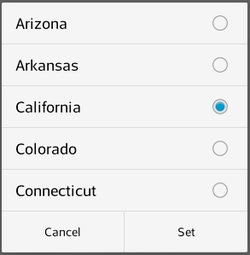The image appears to be a carefully cropped screenshot taken from a phone. The screenshot displays a selection interface with a white background featuring five options arranged in rows. Each row includes the name of a U.S. state in bold black text, accompanied by a circular selection button on the right side. 

1. **Arizona**: Displayed in black text with an unselected circle.
2. **Arkansas**: Displayed in black text with an unselected circle.
3. **California**: Displayed in black text with a circle showing a blue dot, indicating it is selected.
4. **Colorado**: Displayed in black text with an unselected circle.
5. **Connecticut**: Displayed in black text with an unselected circle.

At the bottom of the screen, there are two buttons: one labeled "Cancel" in dark gray text on the left, and another labeled "Set" on the right. The interface suggests making a selection from the listed options, with California currently chosen.